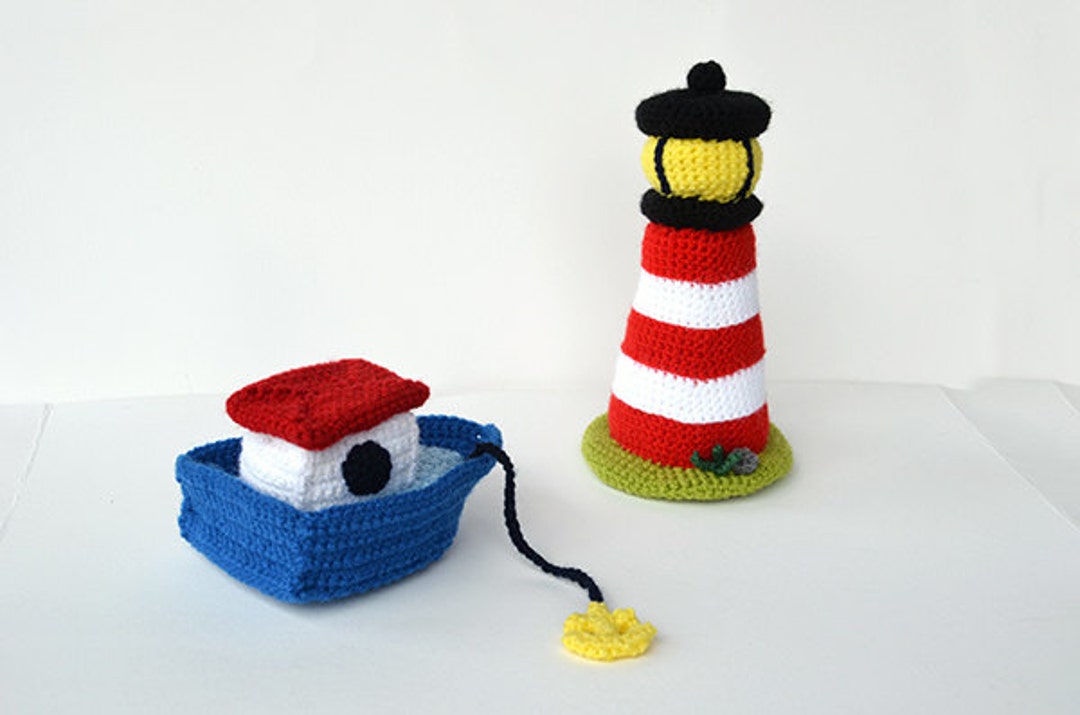In this photograph, set against a light gray background, two detailed crocheted items are showcased on a white table. On the left, there is a small child's toy boat, reminiscent of a tugboat or even Noah's Ark. The boat features a darker blue exterior and a lighter blue interior, with a prominent white deck. At the center of the deck, a black crocheted circle suggests a hole. The boat's roof is a vibrant red, adding a touch of whimsy and warmth to the design.

To the right of the boat stands a meticulously crafted crocheted lighthouse. The lighthouse is striking with its red and white stripes, consisting of three red bands and two white ones, giving it an unmistakable nautical appearance. The lighthouse's base is green, evoking the idea of it being situated on grassy terrain, complete with a darker green crochet detail resembling a shrub. At the top, a black section is capped off with a yellow oval, symbolizing the lighthouse's beacon. Both items, beautifully woven with wool, offer a charming and intricate portrayal of these coastal icons.